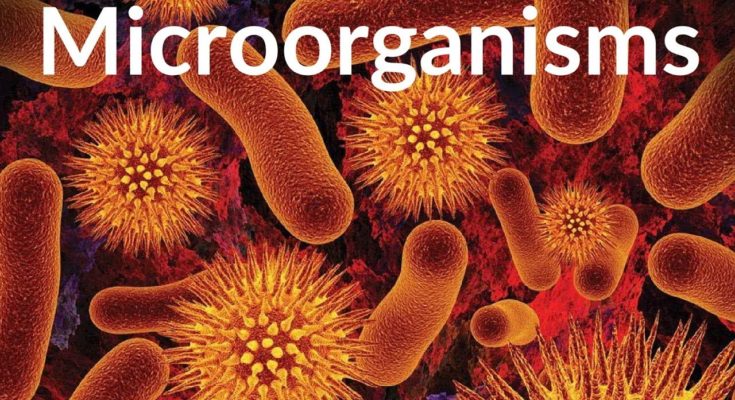The image is a highly detailed, zoomed-in view of a microscopic environment showcasing various microorganisms. Dominating the scene are two distinct types of cells: oval or worm-like tubular structures and spherical cells adorned with spikes extending in all directions. Both types of cells exhibit an orangey-yellow hue. The background is predominantly black, interspersed with out-of-focus red and blue cloud-like structures, enhancing the scientific aesthetic of the image, which is reminiscent of a slide from an educational PowerPoint presentation. The microorganisms are distributed randomly across the image, creating a dynamic and varied composition. At the top of the image, prominently displayed in large white font, is the word "Microorganisms."